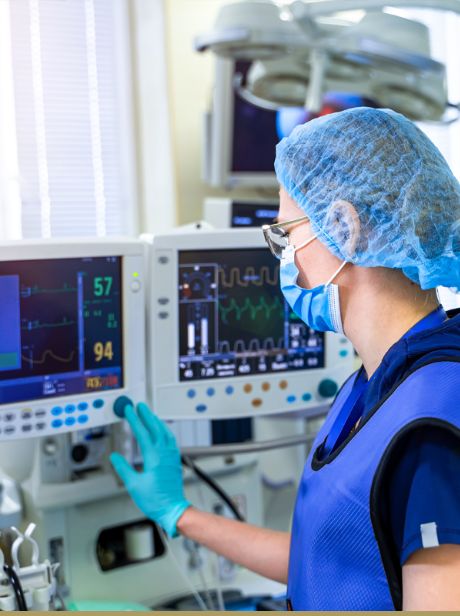The image features a medical professional, likely a nurse, situated on the right side. She is wearing a transparent blue hairnet and glasses, along with a blue medical face mask that covers most of her face. Her attire consists of a dark blue shirt, possibly scrubs, underneath a lighter blue vest. On her right hand, she has a light blue glove, and she is seen touching a large, round dark green button on a device with a display screen. The screen shows various numbers and graphs, including "57" and "94" in green, likely indicating vital signs. Behind this device is another similar screen, both connected to white machinery. The background includes elements that are low-resolution or blurry, including a white door with horizontal slats.